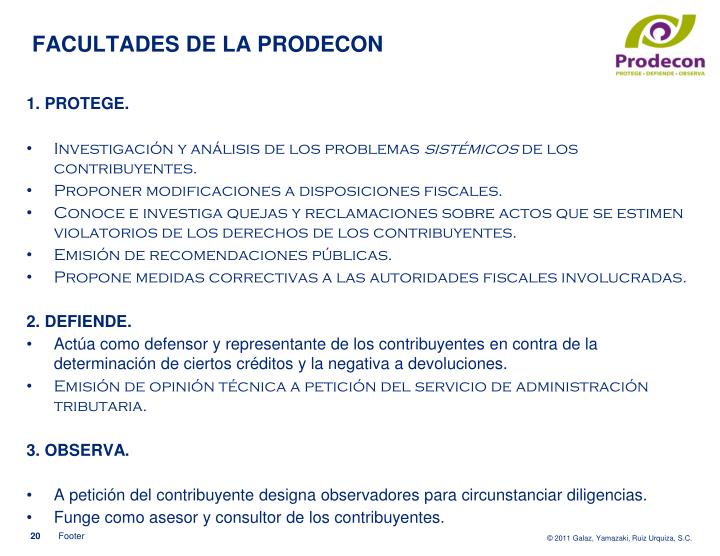This image is a small digital informational card, fully written in Spanish. Dominating the top left corner is a large, striking blue heading that spells "FACULTADES DE LA PRODECON". Adjacent to this, in the upper right hand corner, there's a green and purple logo next to the word "PRODECON" rendered in purple letters, accompanied by some small yellow text below it. The card is divided into three sections.

The first section, labeled "1. Protege", features five bullet points beneath it. The second section, labeled "2. Defiende", has two bullet points, and the third section, labeled "3. Observa", also displays two bullet points. In the bottom corners of the card, there appear to be small numbers accompanied by text, though these details are too miniscule to be clearly discerned.